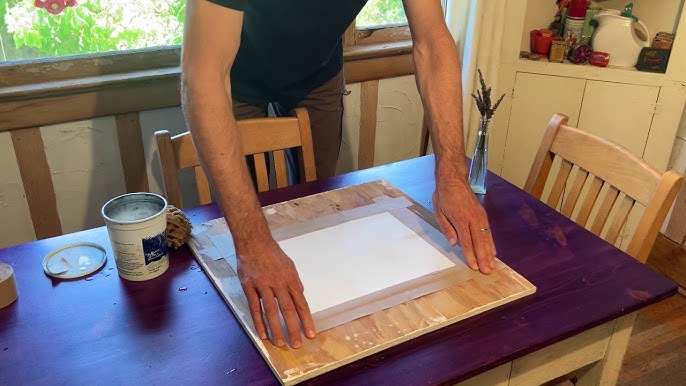In this highly detailed photographic image set indoors, a man is engaged in an art project at a dark-stained kitchen table with a purplish hue. You can only see his torso and arms, which are slightly hairy and wearing a short-sleeved t-shirt and brown pants. His gold wedding ring is noticeable on his left ring finger as his forearms hold down a piece of paper, taped to a square wooden board atop the table. To his left, an open container holds a gray substance, possibly paint, which is complemented by its lid and a natural sea sponge nearby. To the right, a thin glass vase contains a green plant, perhaps an herb. The table, which appears to have visible wood knots, is surrounded by two wooden chairs, one at the head and another in front of the man. Behind the man, a large window reveals greenery outside, including trees and bushes, allowing sunlight to filter in. In the upper right corner of the image, a cabinet with two doors and a nook showcases an assortment of kitchen items, including a Gumby-themed teapot, a white ceramic pitcher, and various jars and cans. The walls feature wainscoting with brown stripes and white textured rectangles in between, and the floor is a dark wood tile, adding warmth to the scene.